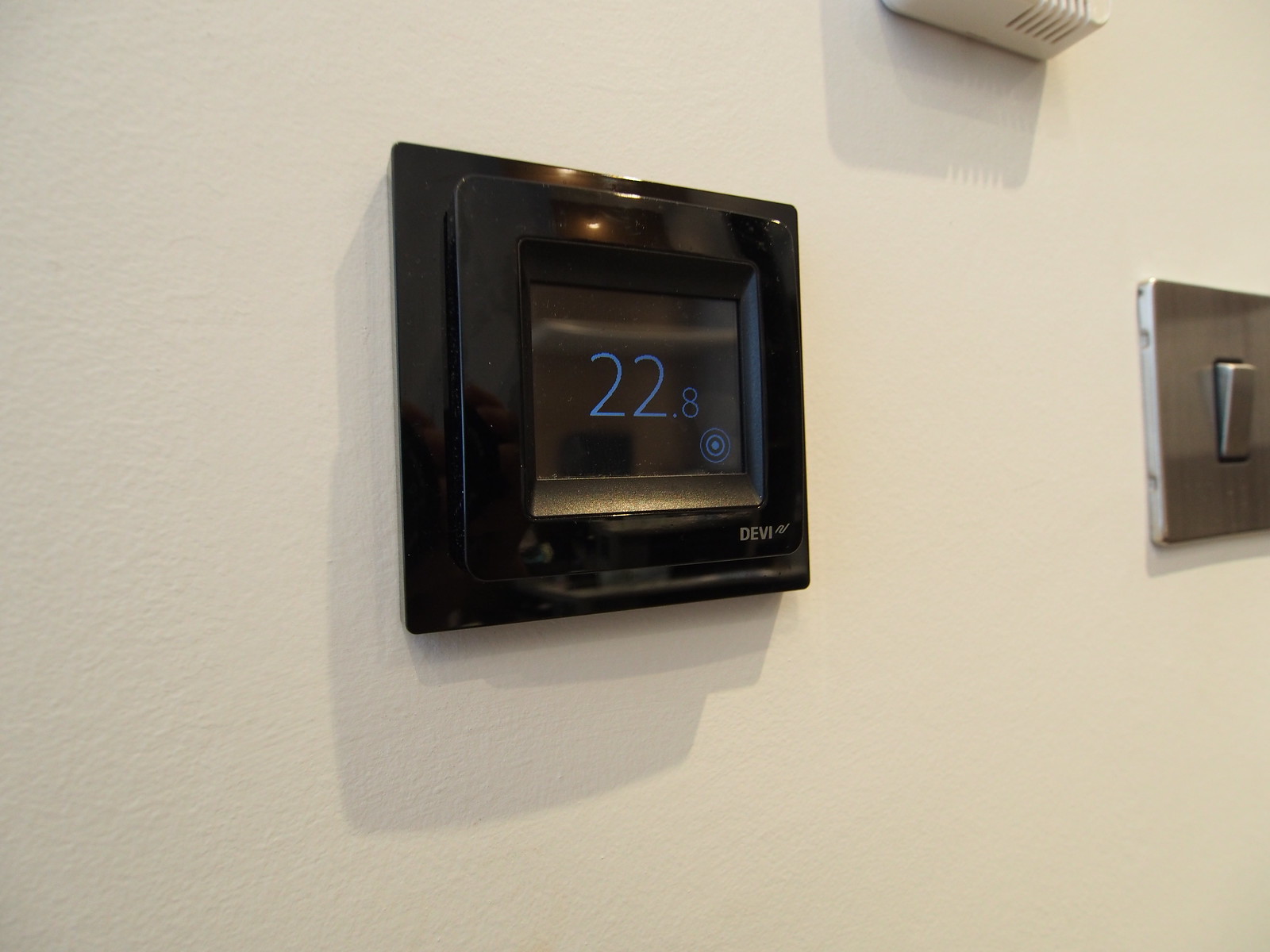In this image, a sleek digital thermostat is centrally built into a white-painted drywall. To the right of the thermostat, there is a modern, silver square light switch featuring a protruding silver push button in the down position, indicating it is off. Above this light switch, a small section of a plastic doorbell unit is faintly visible. The thermostat itself, manufactured by Devi, stands out with its glossy black screen bordered by a black rectangle. The touch screen displays a clear reading of 22.8 degrees in bright blue numbers. Below the temperature display, there are nested blue circle icons, possibly indicating additional features or settings. This sophisticated device integrates seamlessly into the wall, demonstrating its high-tech functionality and modern design.